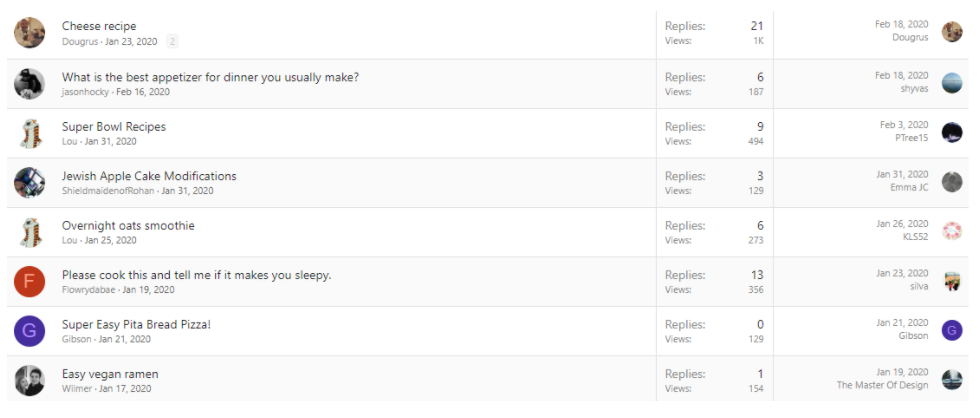The image showcases a detailed list of posts from a forum, each accompanied by the number of replies and views. The posts are organized in two columns. The left column features the titles of the forum threads as follows:

1. "Cheese Recipe" 
2. "What is the Best Appetizer for Dinner You Usually Make?"
3. "Super Bowl Recipes"
4. "Jewish Apple Cake Modifications"
5. "Overnight Oats Smoothie"
6. "Please Cook This and Tell Me If It Makes You Sleepy"
7. "Super Easy Pita Bread Pizza"
8. "Easy Vegan Ramen"

The right column lists the engagement metrics for each post:

1. "Cheese Recipe" - 21 replies, 1k views
2. "What is the Best Appetizer for Dinner You Usually Make?" - 6 replies, 187 views
3. "Super Bowl Recipes" - 9 replies, 494 views
4. "Jewish Apple Cake Modifications" - 3 replies, 129 views
5. "Overnight Oats Smoothie" - 6 replies, 273 views
6. "Please Cook This and Tell Me If It Makes You Sleepy" - 13 replies, 356 views
7. "Super Easy Pita Bread Pizza" - 0 replies, 129 views
8. "Easy Vegan Ramen" - 1 reply, 154 views

This well-organized forum list provides an overview of popular culinary topics alongside their community engagement levels, offering a snapshot of current discussions and interests.